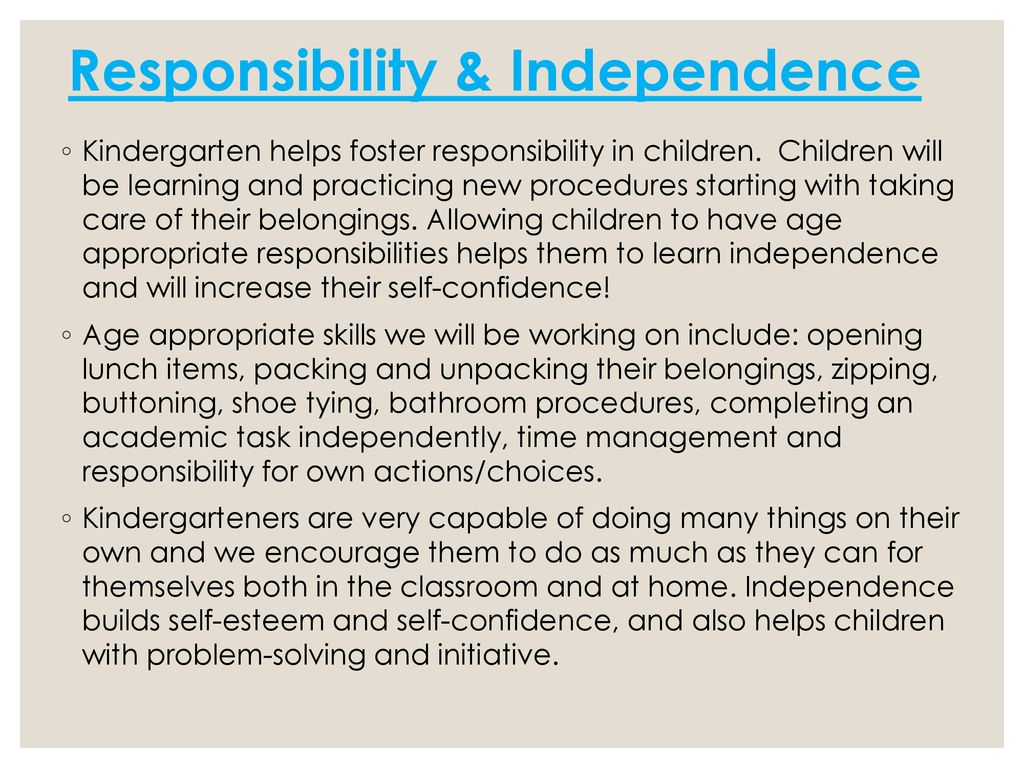The image features a slide with a title at the top in bold, light blue font that reads "Responsibility and Independence," and is underlined in blue. Below the title are three detailed bullet points in black font. The first bullet point explains how kindergarten helps foster responsibility in children by teaching and practicing new procedures, such as taking care of their belongings. It emphasizes that allowing children to have age-appropriate responsibilities aids in learning independence and boosts their self-confidence. The second bullet point lists specific age-appropriate skills that will be developed, including opening lunch items, packing and unpacking belongings, zipping, buttoning, shoe-tying, bathroom procedures, completing academic tasks independently, time management, and taking responsibility for their own actions and choices. The third bullet point highlights that kindergartners are capable of many tasks independently and encourages them to do as much as possible on their own, both in the classroom and at home. It further explains that independence builds self-esteem, self-confidence, and enhances problem-solving skills and initiative. The slide is presented on a beige background with small black circles as bullet points.